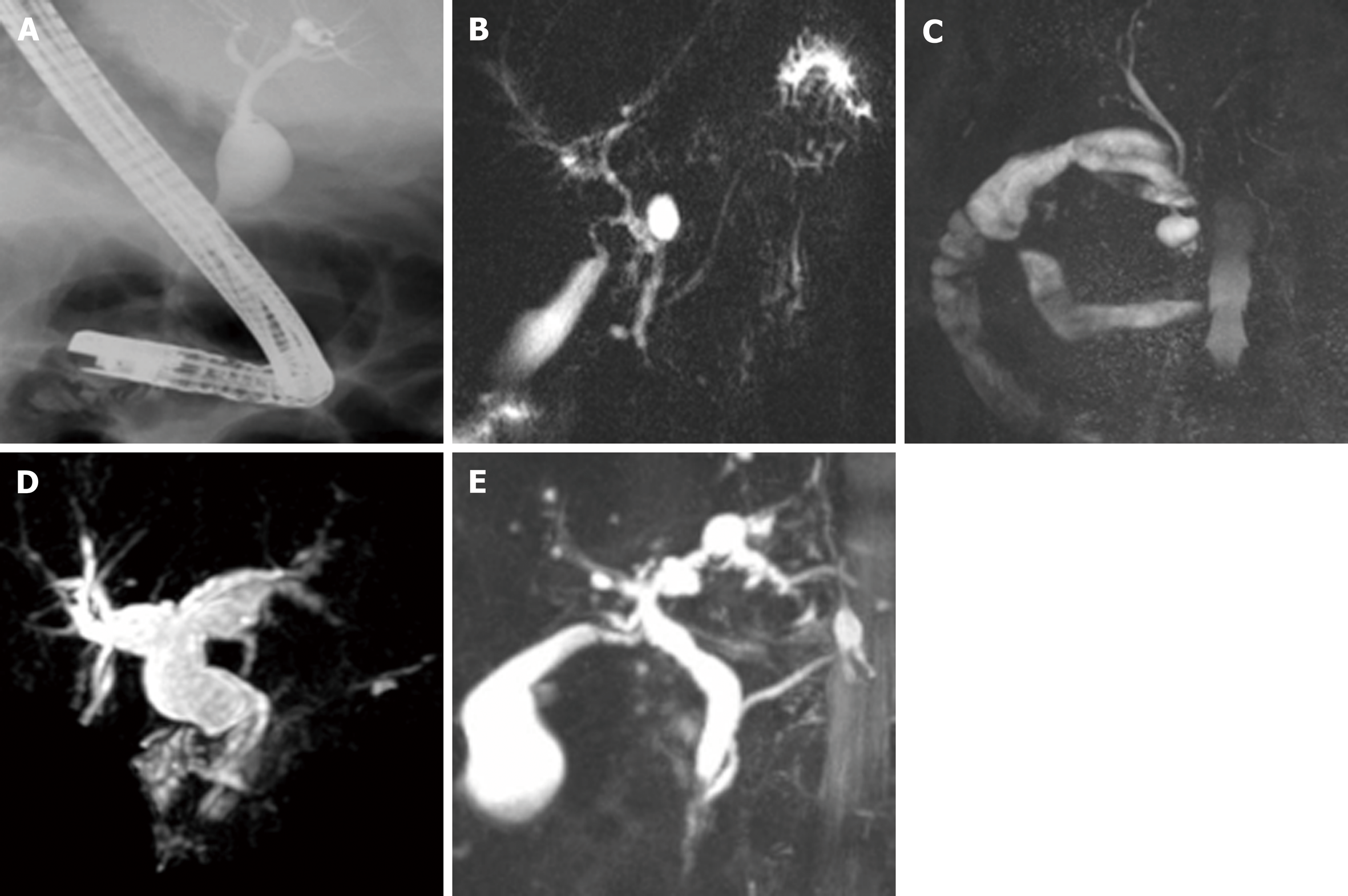The image presents a series of five black-and-white photographs, labeled A through E, showcasing various organic forms that resemble medical specimens or slides. Each image is set against a dark, cloudy, or foggy background, creating a stark contrast with the bright, detailed organisms.

In image A, situated at the top left, a smoky, white, straw-like organism bends towards the right, reminiscent of an L-shape, with a bulbous structure behind it. Image B displays a darker backdrop featuring a white, vein-like structure with appendages extending from its sides, and rounded formations connected by thin lines or veins.

Image C reveals a creature that resembles an arthropod or a small shrimp, with observable limbs and antennae, set against a grayish background. In image D, a triangular white organism with numerous small tendrils or spokes radiating from its body is centrally positioned on a black background, its shape somewhat abstract and less recognizable.

Finally, image E features a larger, bulbous-limbed organism within a grayish-black background, detailed with several pronounced limbs and darker sections at the top, creating a vivid and intriguing visual composition.